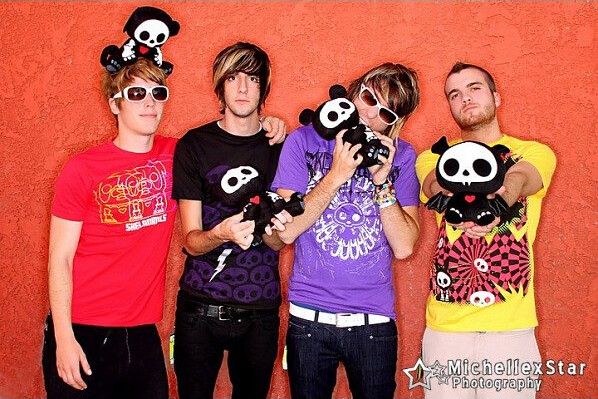In this colorful and lively professional photograph by Michellex Star Photography, four young men, likely in their late teens to early twenties, stand against a vibrant reddish-orange background, exuding a playful, band-like energy. From left to right, the first young man is wearing a red t-shirt with an abstract white pattern and text, paired with black jeans. He is notably holding a plush toy that resembles a panda, characterized by its white face, black eyes, triangle black nose, red heart on its chest, and white markings on its feet. This young man also has shaggy hair with blonde streaks and white-framed sunglasses.

Next to him, the second individual, slightly taller with long side-swept bangs and dark hair, sports a black t-shirt adorned with a purple version of the same panda-like face found on the toy they are all holding. Moving along, the third young man is clad in a bright purple t-shirt and blue jeans, characterized by his action of biting the plush toy, which adds an element of playful mischief to the scene. He, too, wears white-framed sunglasses.

Lastly, the fourth individual stands out with his shorter hair and beard, dressed in a yellow t-shirt featuring a red and black checkerboard spiral pattern, again incorporating images of the panda-like creature. He complements his outfit with white jeans. This group, with their distinct yet harmonious appearances, and the recurring motif of their unique toys, could easily be perceived as a band or part of an ensemble for a kids' show, captured vibrantly in this professional shot.